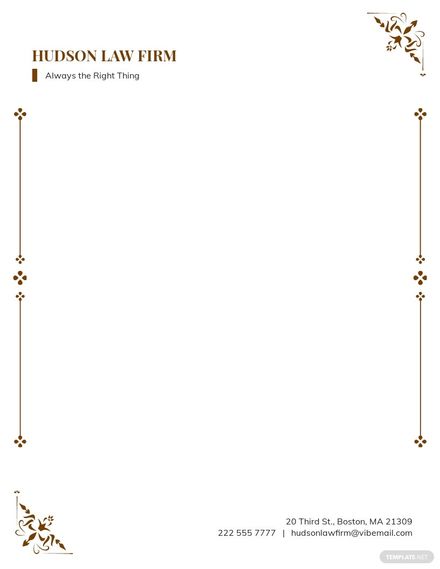The image depicts a detailed and elegantly designed letterhead for Hudson Law Firm. The top left corner prominently features "HUDSON LAW FIRM" in bold, all-capital brown text. Directly below, a small brown dash separates the firm's slogan in smaller black text: "Always the Right Thing." Decorative elements adorn the top right and bottom left corners, consisting of elaborate angled flourishes. The borders on both sides of the letterhead include vertical rules embellished with a four-cluster blossom at the center and at each end. The bottom right corner lists the firm's contact information in black text: "23rd Street, Boston, Massachusetts, 21309," followed by the phone number "222-555-777" and the email "HudsonLawFirm@vibemail.com." Additionally, there is a gray, pill-shaped badge at the bottom right, possibly reading "Template" or "Template.net," indicative of the template's origin. The frame surrounding the entire letterhead features lines with three little dots, enhancing the sophisticated aesthetic of the design.